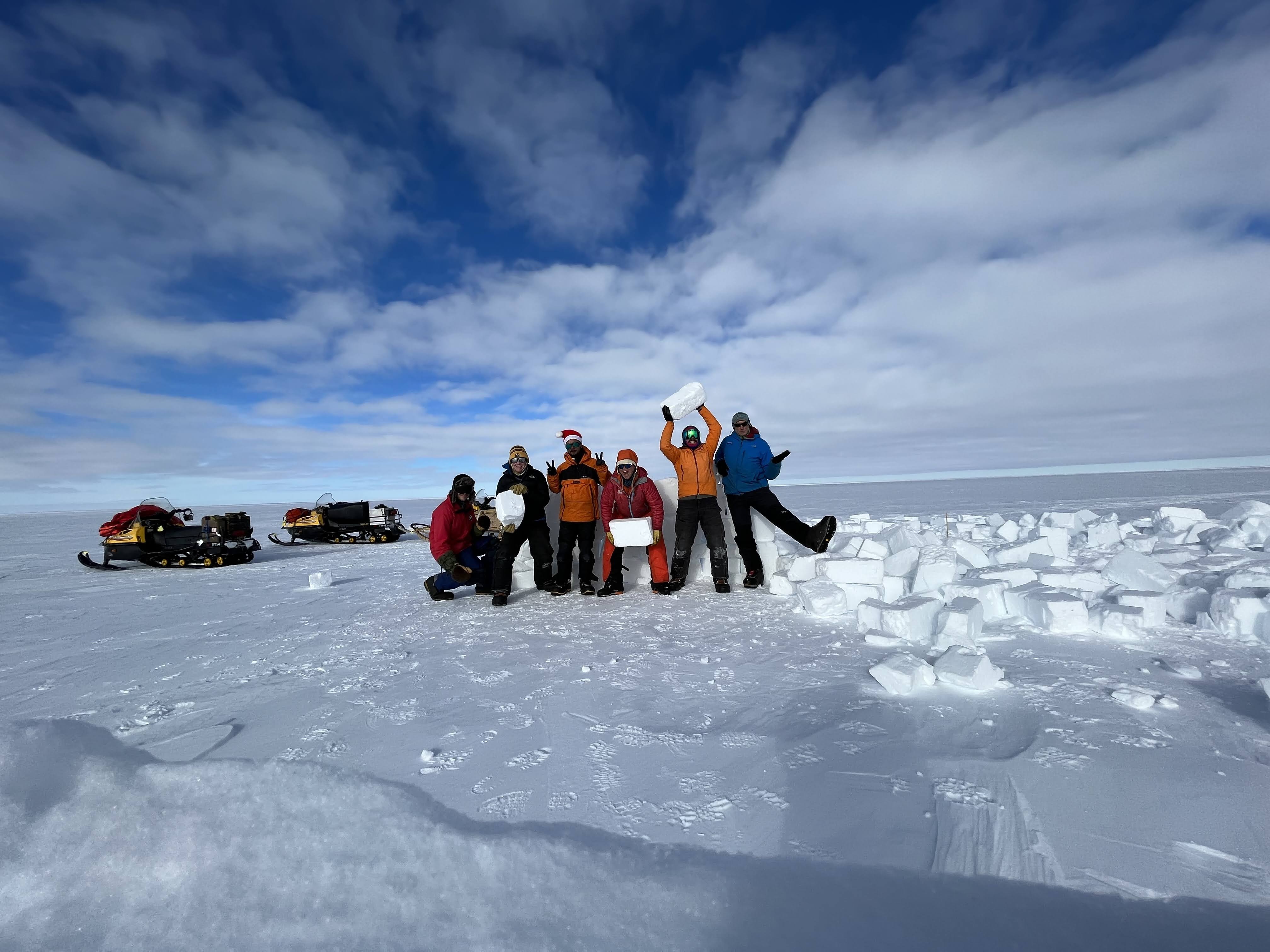In a vast, frozen landscape, likely a body of water covered in snow and ice, six people stand posed for a photograph. Dressed in a variety of brightly colored winter clothing, including jackets in red, yellow, and blue, black jeans, and protective gear like beanies and sunglasses, these individuals appear to be men, with some sporting Santa hats for a festive touch. They stand about 20 feet from the camera, holding large rectangular ice blocks, while a nearby pile of similar blocks sits to their right. Two snowmobiles, primarily black with yellow accents, are parked to the left of the group. Above them, the sky is a mix of blue patches and white clouds, illuminated by broad daylight. The scene exudes a chilly yet lively atmosphere, characteristic of an adventure in remote icy regions such as Antarctica or Alaska.